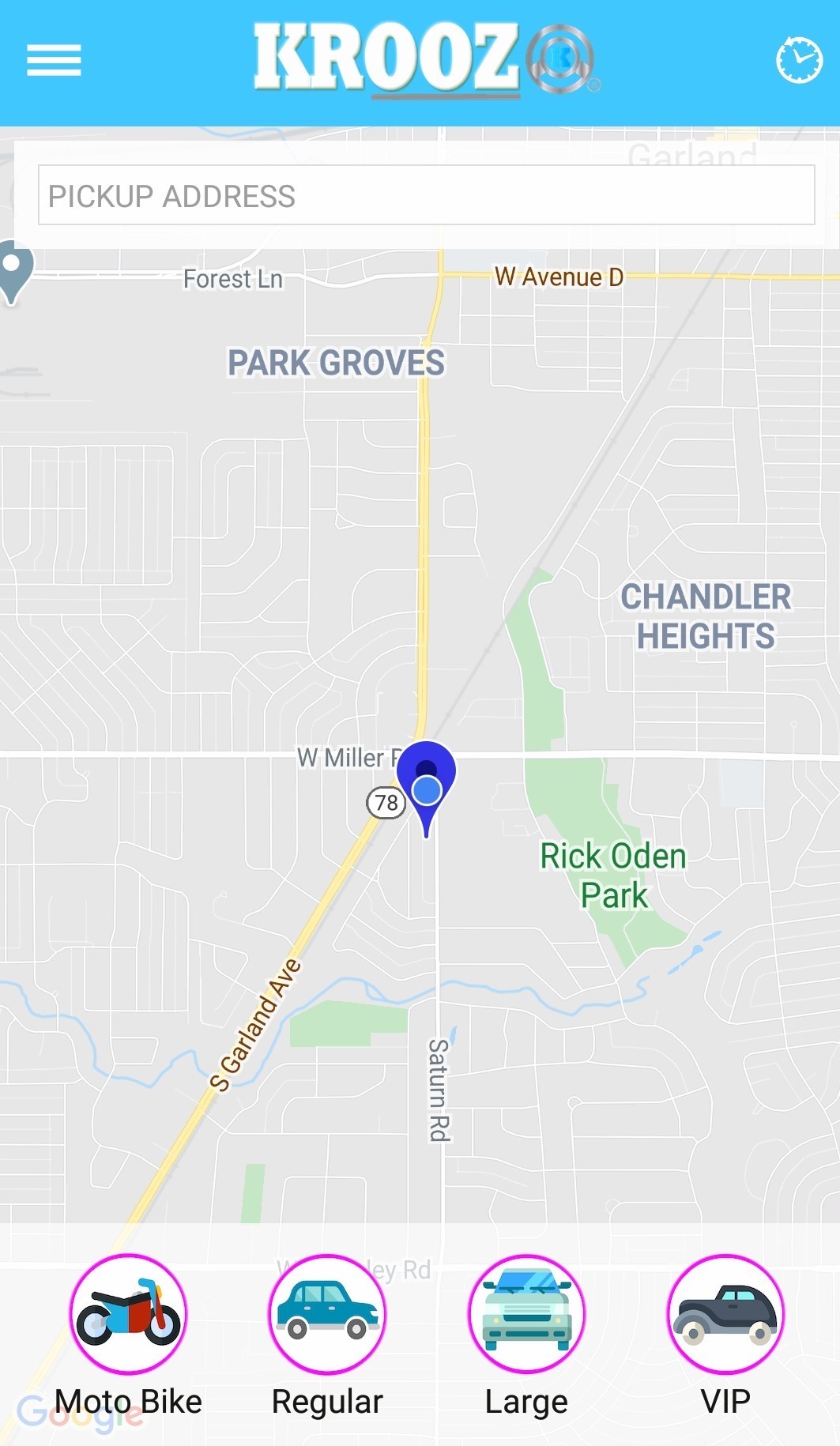In the image, the top section showcases the label "KROOZ" in white text against a blue background. Below this, the blue background continues, featuring three horizontal lines on the left and a clock icon on the right. Directly beneath, there's a white box with the text "PICK UP ADDRESS" in all caps on the left side. Below this box, a map is displayed, detailing several city and road names, including "S. Garland Avenue," "Park Road" (mentioned twice), and "Chandler Heights." A notable landmark on the map is "Rich Oden Park," highlighted in green. Prominently positioned in the center of the map is a blue pinpoint marker encircled by a blue ring. At the bottom of the image, four circular icons depict different types of vehicles. From left to right, these circles feature: a motorcycle labeled "Motorbike," a blue car labeled "Regular," another car labeled "Large," and a black car labeled "VIP."